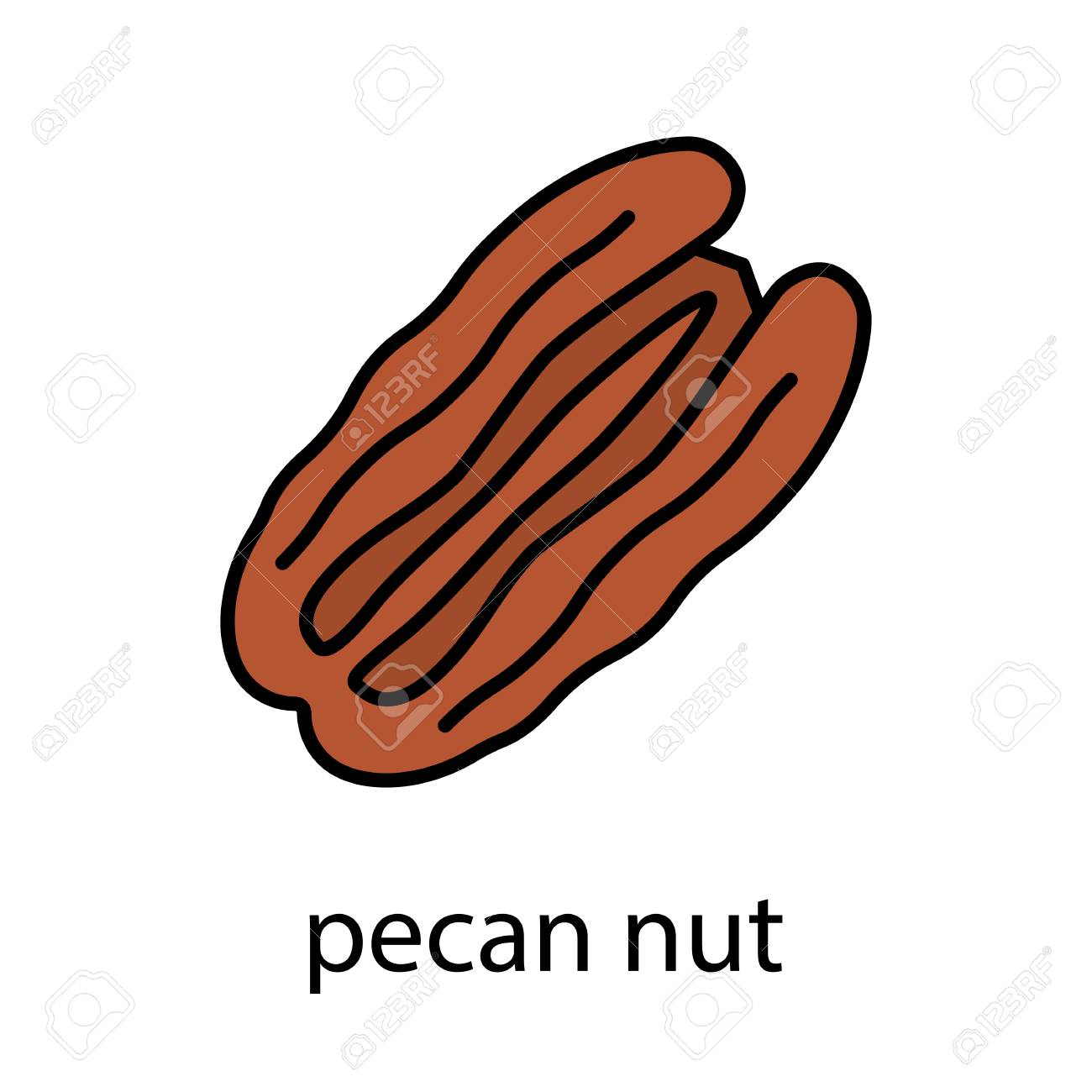The image features a detailed clipart depiction of a pecan nut against a solid white background, which is interspersed with alternating sketches of a camera and the icon "123RF" as a watermark. The pecan nut is illustrated using thick black lines to accentuate its grooves and contours, rendering it in a rich mocha brown color. Below this central figure, the label "pecan nut" is succinctly printed in lowercase black letters. Despite its misshapen appearance, the identifying label underscores the nut's identity, offering clarity that might otherwise be obscured by its abstract representation. Overall, it appears to be a stock photo aimed at showcasing the pecan nut's shape and structure.